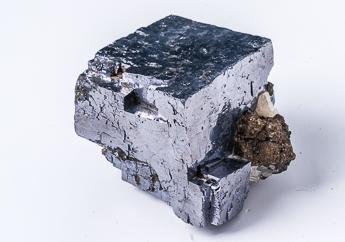This photograph features a metallic silver rock or mineral with distinct angular and flat planes, creating a roughly square shape at the top that narrows into a more irregular form towards the bottom. The rock is situated on a plain white background, casting light shadows to the right side. Notably, attached to the right side of the metallic silver rock is a contrasting segment composed of a bronze or dark brown substance with hints of tan, resembling either dirt or a sandy texture. On top of this segment, there is a white, pearly mineral. The rock overall has rough edges and an uneven surface, though it maintains a reflective, shiny finish.